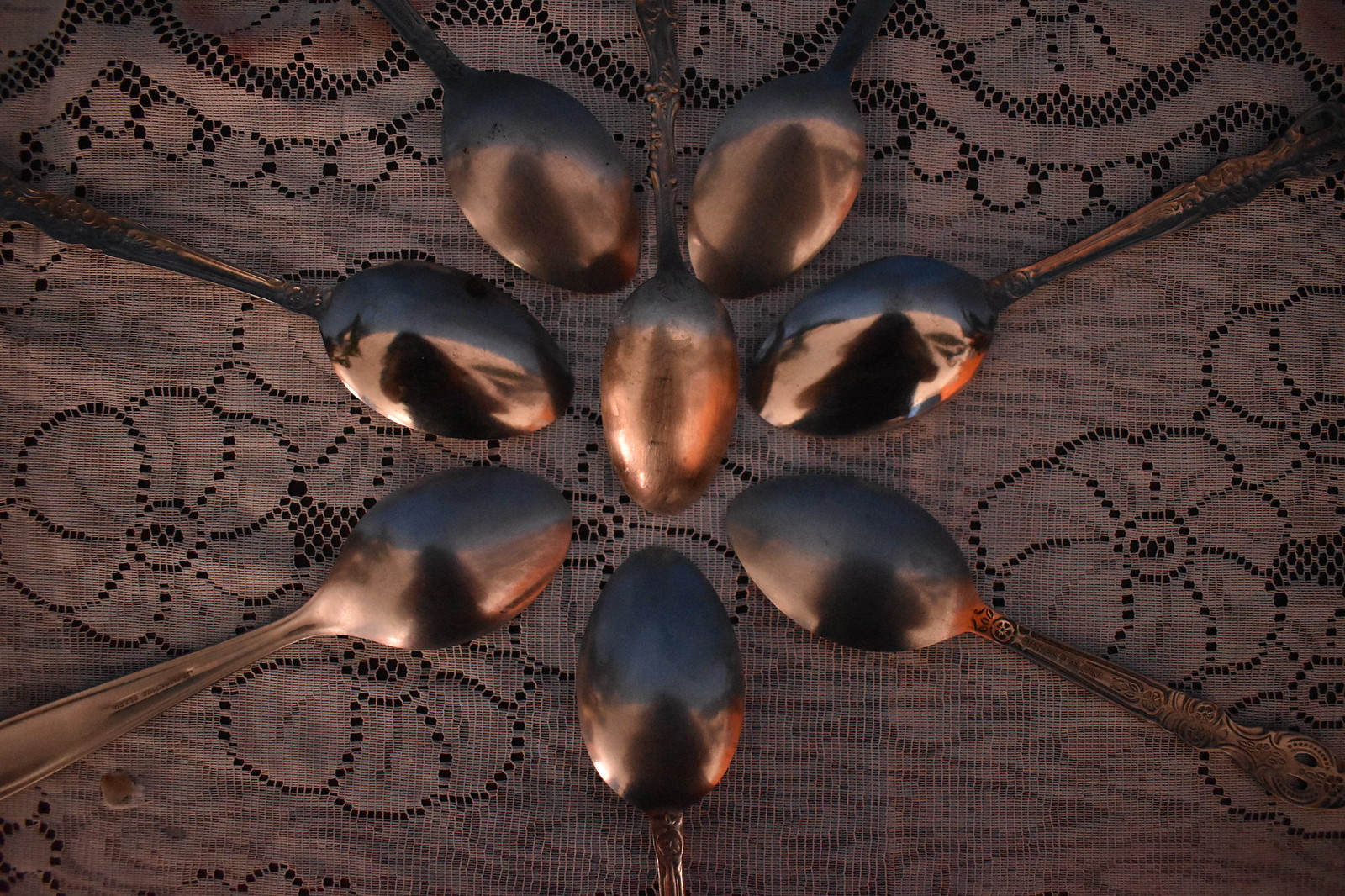This is a semi-professional photograph set in a dimly lit room with a dark ambiance. The focus is on a carefully arranged composition of eight metal spoons, placed on a table covered with an ornate white lace tablecloth featuring a floral pattern. The spoons, which have an antique patina and ornate handles, are arranged in a circular pattern with their backs facing up, creating a flower-like design. One spoon extends into the center of this circle, forming a focal point. The reflective surfaces of the spoons capture the shadowy silhouette of the photographer, likely a woman with long hair, who appears blurred and indistinct due to the low light. This detailed arrangement and the interplay of antique aesthetics and soft reflections convey a sense of warmth and subtlety in the image.